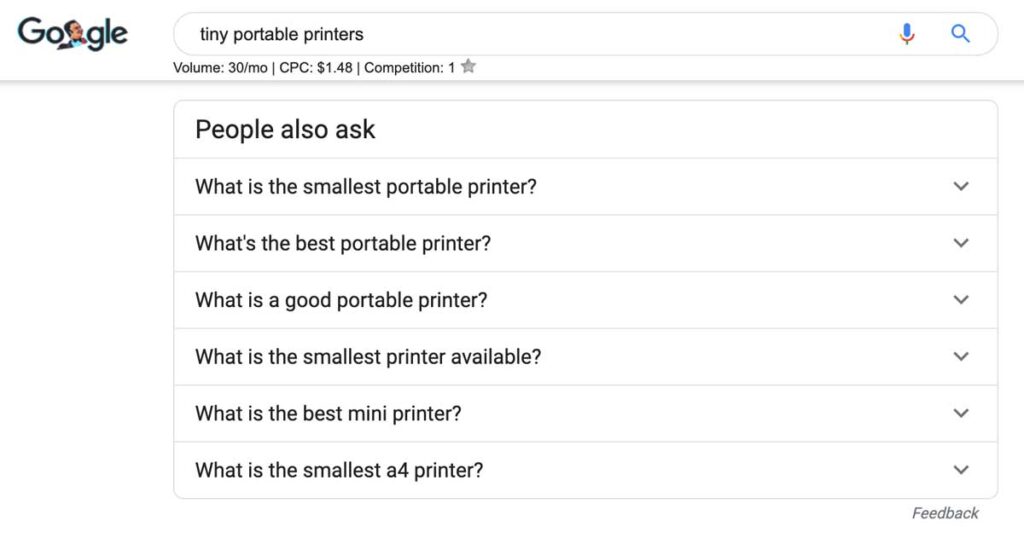A detailed caption for the described image:

The screenshot depicts a Google search results page on a computer. In the upper left corner, the word "Google" is displayed in black. Replacing the second "O" in Google is a small avatar or picture of a man. The search query "tiny portable printers" is entered in the search bar at the top of the screen. To the right of the search bar are a blue magnifying glass icon and a microphone icon. Below the search bar, the "People also ask" section is displayed, featuring a series of expandable questions related to portable printers. The questions listed are:
- What is the smallest portable printer?
- What is the best portable printer?
- What is a good portable printer?
- What is the smallest printer available?
- What is the best mini printer?
- What is the smallest A4 printer?

Each question has a small down arrow to its right, indicating that users can click to reveal the answers. At the bottom right corner of the image, the word "feedback" is visible. The image is mainly composed of the search bar, the list of questions, and their interactive elements, without a defined border or surrounding rectangle.